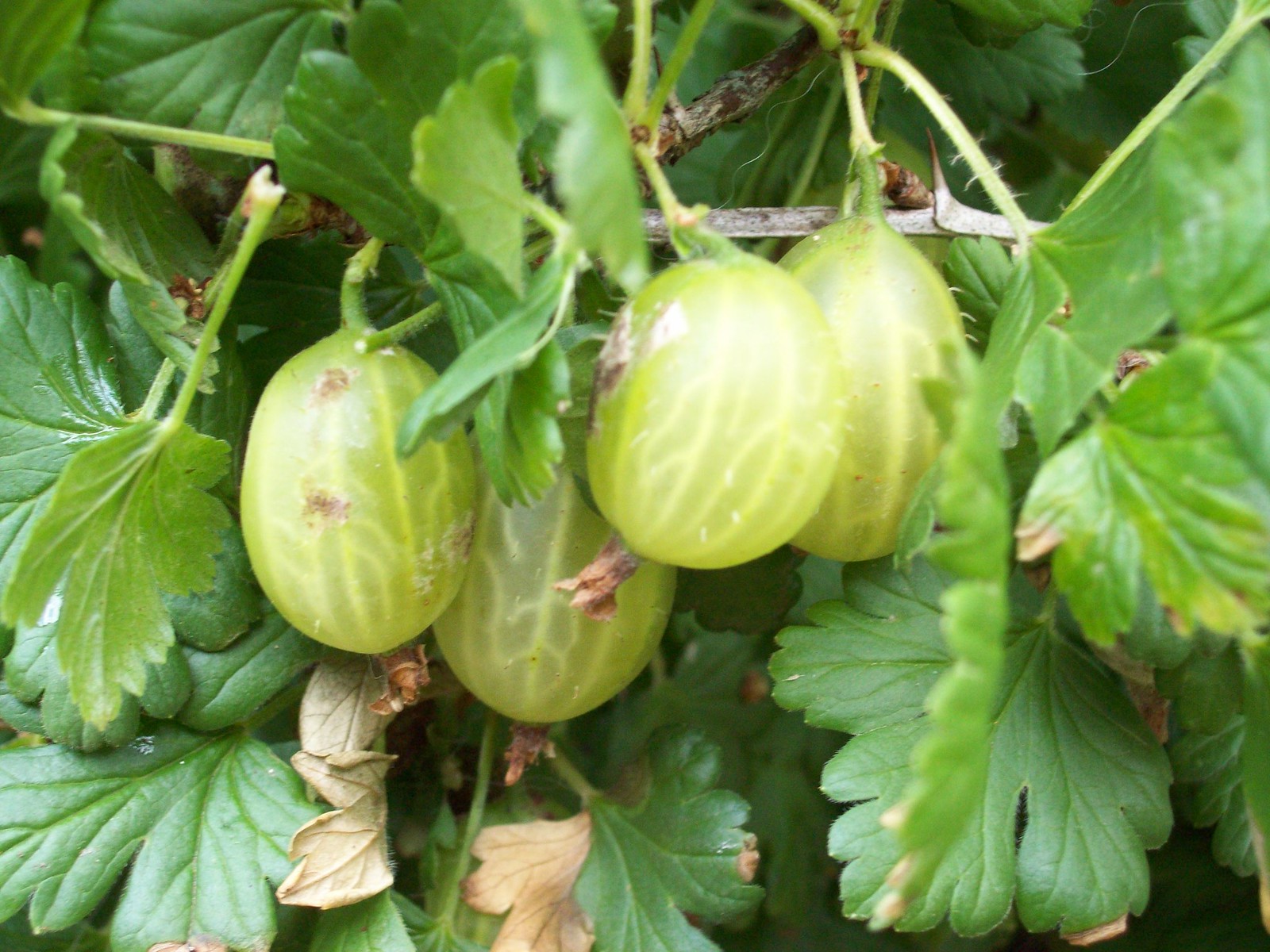The image is a detailed close-up of a cluster of small, green fruits that closely resemble gooseberries. These four oval-shaped fruits, similar in size to grapes but slightly larger, are characterized by vertical tan and white vein-like lines on their skins. A couple of the fruits have noticeable brown spots. The fruits are still attached to their green stems, which connect to a larger brown branch that curves across the top of the image. This branch also features small thorns. Surrounding the fruits are lush green leaves, some of which are bright and healthy, while others show signs of browning or withering. In the background, blurred lighter green leaves can be observed. The overall composition highlights the natural textures and intricate details of the fruit and foliage.